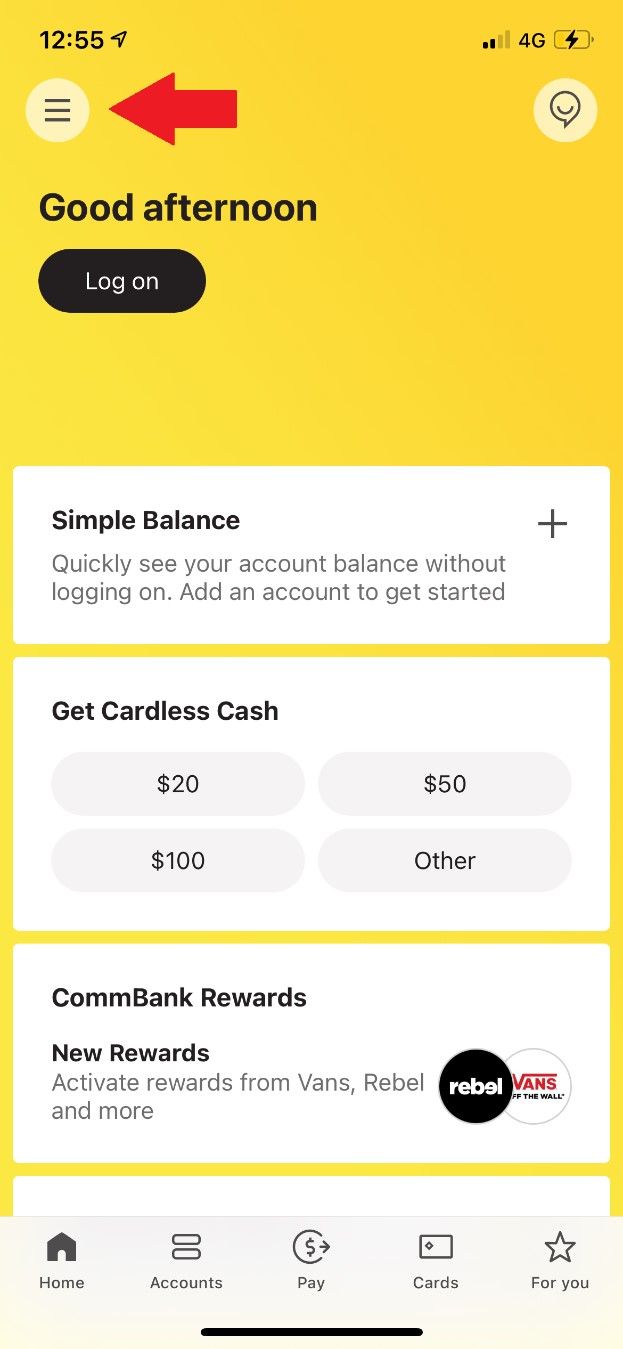A screenshot captures a mobile banking application interface displayed on a phone at 2:55 PM, as indicated in the upper left-hand corner. The upper right-hand corner shows that the phone is connected to Wi-Fi, has a 4G connection, and is currently charging. The app's background is a bright, sunny yellow.

In the upper left-hand corner of the app, a navigation button can be seen, highlighted by a bright red arrow that has been edited onto the screenshot. This button is designed to open a side tab for easier navigation. In the upper right-hand corner, there's another button resembling a speech bubble with a smiley face inside.

The app's welcome message, "Good Afternoon," is displayed in black text on the left side, with a "Log On" button directly beneath it. The interface features several white boxes below the greeting. The first box offers a "Simple Balance" option, allowing users to quickly view their account balance without logging on by adding an account. This box includes a small plus sign. 

The second box is labeled "Get Cardless Cash," providing options for withdrawing set amounts of $20, $50, $100, or a customizable 'Other' amount. Further down, the "ComBank Rewards" box advertises new rewards and includes logos from brands like Vans and Rebel to indicate available offers. 

Partially visible below the rewards box is another section, which requires scrolling to view fully. Spanning the bottom of the screen are navigation buttons labeled Home, Accounts, Pay, Cards, and For You, providing easy access to the main functions of the app.